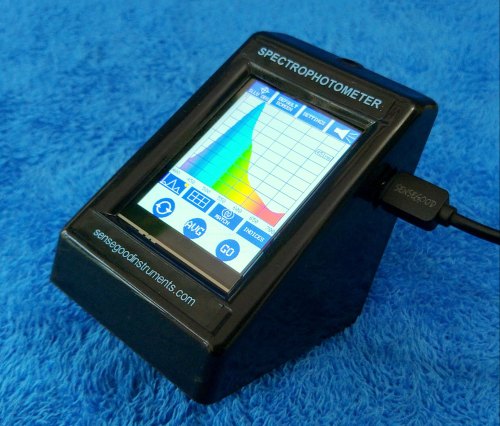A black spectrophotometer, labeled "N-White Spectrophotometer" at the top and "SenseGoodInstruments.com" at the bottom, rests on a plush blue carpet. The device has a screen in the middle displaying a rainbow-colored graph transitioning from purple, blue, green, yellow, orange, to red on the right-hand side. The graph is flanked by blue boxes at the top and bottom and three blue circles at the screen's bottom. The instrument, centrally placed in the image, has a cord plugged into its right-hand side, with the cord trailing off the image. The overall setting appears to be a domestic environment.